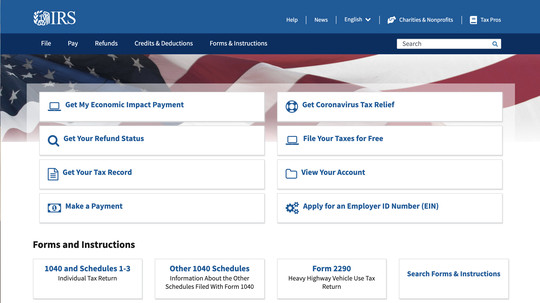In this image, we see a meticulously captured screenshot of a website that appears to be the IRS homepage. The layout is wide, emphasizing the website's horizontal orientation. The topmost part of the screen is marked by a blue header. Positioned on the upper left corner, the IRS logo is prominently displayed in white, accompanied by the text "IRS."

On the right side of the header, a navigation menu includes the following options: "Help," "News," "English" (with a drop-down menu for language selection), "Charities and Nonprofits," and "Tax Pros." Directly beneath this section, a dark blue banner stretches across the width of the screen, featuring white text links that read: "File," "Pay," "Refunds," "Credits and Deductions," "Forms and Instructions," and a prominently placed white search bar.

The central section of the screen is occupied by a partly visible image of the American flag, rendered in shades of red, white, and blue. The flag appears to be waving, with the white stars situated on the upper left side and the red and white stripes extending to the right.

At the bottom portion of the screen, bold black text prominently displays the section title: "Forms and Instructions." Immediately below this, a row of buttons is neatly arranged, labeled from left to right as follows: "1040 and Schedules," "Other 1040 Schedules," "Form 2290," and "Search Forms and Instructions."

The website design is visually structured to guide users efficiently through various IRS services and forms.